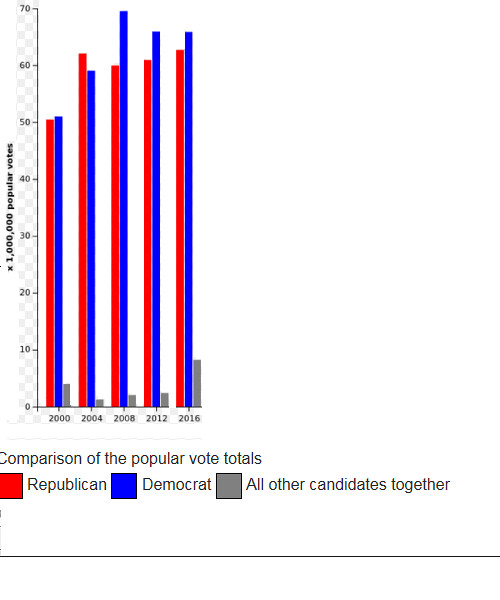The image is a detailed bar chart representing the popular vote totals for different election years, focusing on the comparison between Republicans, Democrats, and all other candidates combined. At the bottom of the chart, there is a legend with a red box for Republicans, a blue box for Democrats, and a gray box for all other candidates together. Horizontally, the chart is labeled with the years 2000, 2004, 2008, 2012, and 2016. Vertically, the chart is labeled "X, 1 million popular votes," and the scale ranges from 0 to 70 million votes in increments of 10 million. The bars are colored red, blue, and gray respectively and rise according to the popular vote totals for each election year.